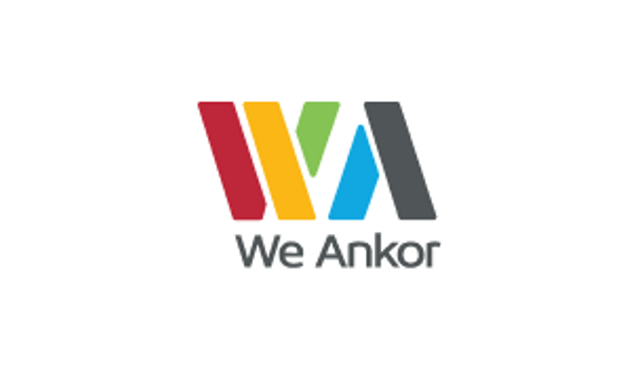The image is a graphic logo set against a completely white background. The logo, which spells out "WE ANCOR" in grey text, is composed of various colored elements that form stylized letters resembling "W" and "A." The "W" consists of two parallel bars, one red and one orange, slanting diagonally from the top left to the bottom right. Crossing these is a shorter green bar, slanting from the bottom left to top right. The "A" is represented by a blue diagonal bar running from the center to the top right and a longer dark grey bar extending from the top right to the bottom left. Below the logo, in the same grey color as the letters, is the text "WE ANCOR," with the letters W-E-A-N-C-O-R clearly spelled out.